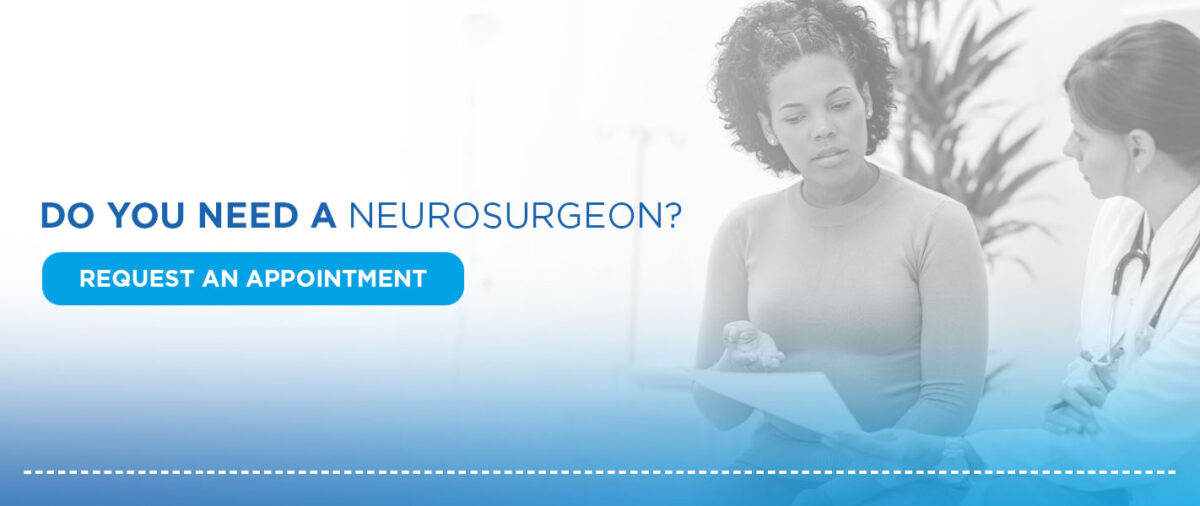The image appears to be an online web page for a neurosurgeon's office. On the right side, there's a grayscale-tinted photograph of a doctor and a patient. The doctor, wearing a white lab coat and a stethoscope around her neck, has dark hair tied back and is holding a piece of paper in her left hand. She also has a pen between the fingers of her right hand and wears a watch on her left wrist. The patient, with dark hair pulled back and wearing earrings and a form-fitted, light-colored long-sleeved top, is gesturing towards the paper that the doctor is holding. Behind them, a plant is visible, adding to the office setting.

On the left side of the image, a white background features blue text that reads, “Do you need a neurosurgeon?” Below this, there is a blue rectangular button with rounded corners and white text that says, “Request an appointment.” The bottom of the photo fades into a blue tint with a dashed white line running across its length, adding a cohesive aesthetic touch. This composition gives the impression of an inviting and professional portal for patients seeking neurosurgical consultations.